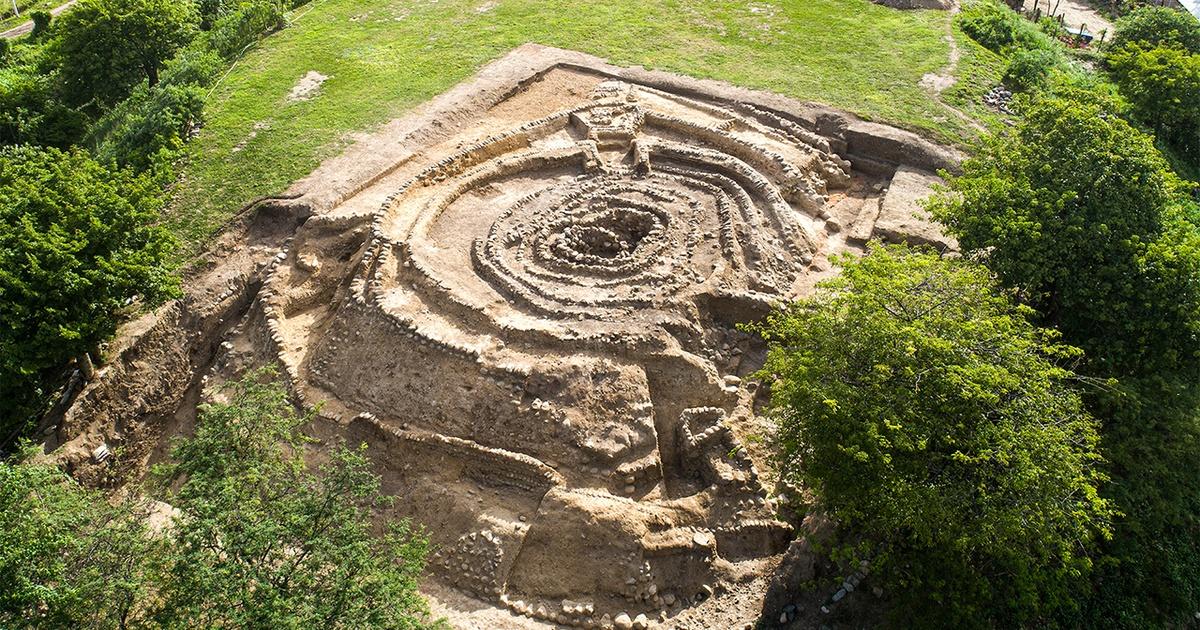The aerial photograph captures a decrepit, ancient fort-like structure nestled in a verdant landscape, surrounded by dense greenery on three sides and open green lawns on one side. The structure, characterized by its earth-tone sandy hues, seems to be centuries old and heavily worn, with various parts crumbling and rocks scattered on the ground. This abandoned relic, potentially from Amazonian times, features multi-levels and strategic openings, possibly for defense, reminiscent of an old fort used for protection. Intriguingly, a winding path or swirly line leads to a prominent hole in the top center of the structure, adding to its mysterious allure. Amidst the encroaching wilderness, three bushes stand out on the right side, their foliage displaying rich shades of forest and emerald green. The image also reveals another sandy patch on the top right, hinting at a pathway that interconnects different parts of this historic site.